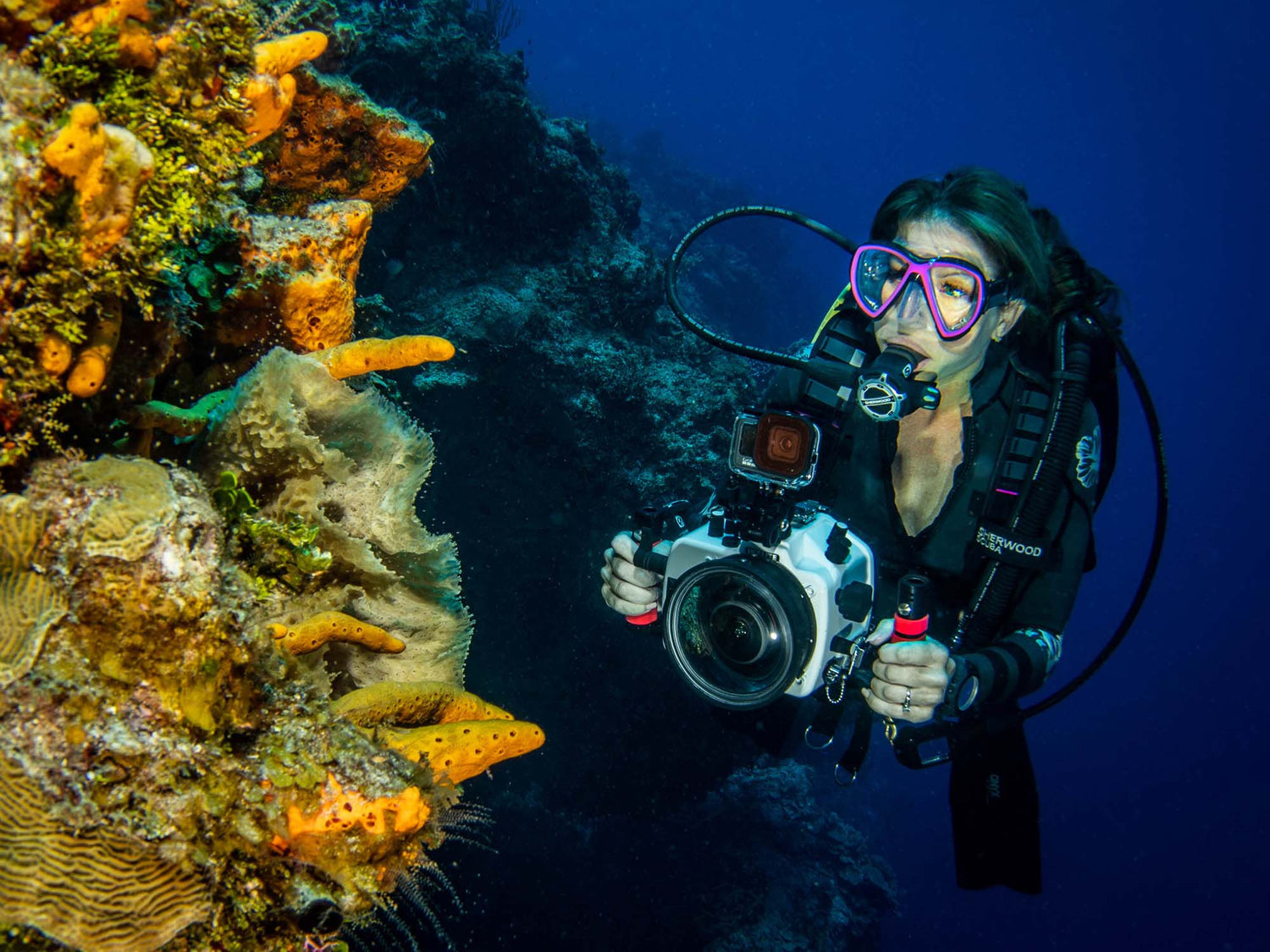This underwater photograph captures a female diver in a black wetsuit holding a large, professional camera with dual grips featuring black and red stripes. She is equipped with scuba gear, including a black respirator and a purple and black mask lined with pink. Her black flippers are also visible. The diver is positioned slightly to the right, swimming in a deep blue ocean. To her left, vibrant coral formations dominate the view, featuring striking colors such as vivid oranges, yellows, greens, and aqua tones. The coral has detailed projections and black-dotted orange segments, contrasting with some darker, possibly dead coral or rocks in the background. The overall scene is rich in color and detail, showcasing both the diver's equipment and the surrounding underwater environment.